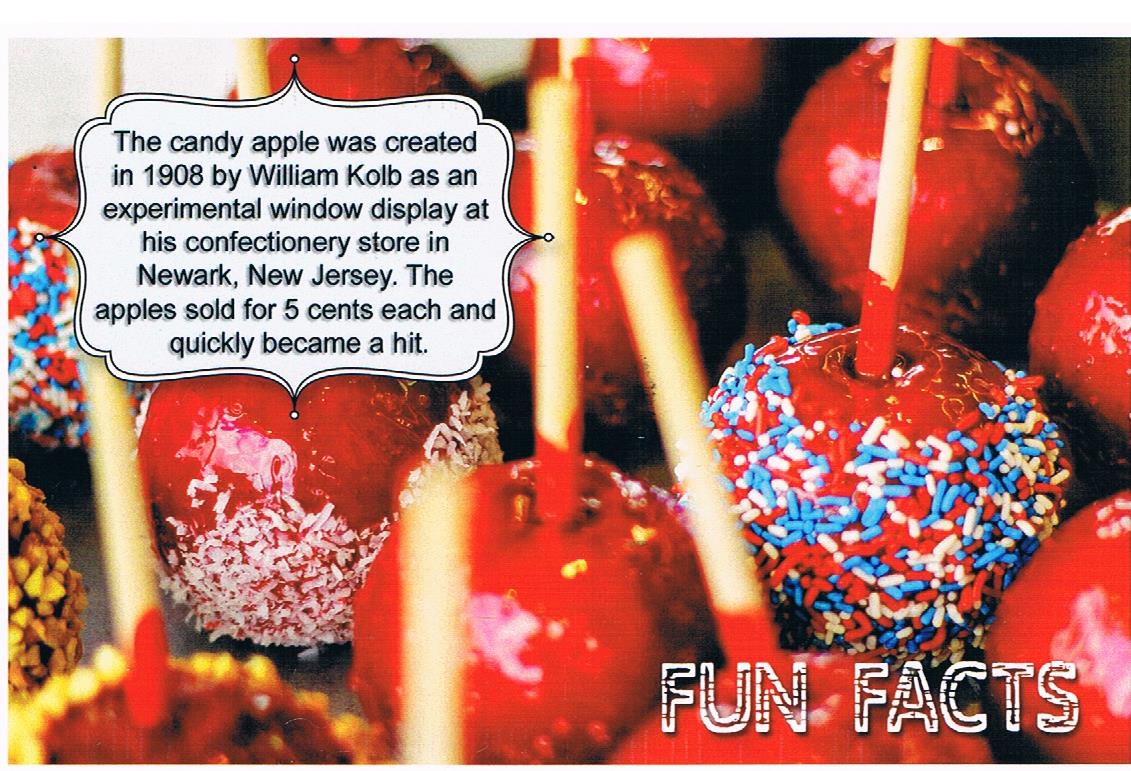The image showcases a vibrant assortment of candy apples that dominate the frame, with sticks protruding from the top of each apple, suggesting they’ve been freshly coated and left to dry. These candy apples are richly decorated with a variety of toppings: some have red, white, and blue sprinkles, others are adorned with plain white sprinkles or gold flake-like toppings that might be coconut. Additionally, several of the apples are covered simply with the shiny, red candy coating, highlighting the diverse range of decorative styles.

In the upper left corner of the image, a dialog box with a white background and shadowed black sans-serif text provides historical context: “The candy apple was created in 1908 by William Kolb as an experimental window display at his confectionery store in Newark, New Jersey. The apples sold for five cents each and quickly became a hit.” In the lower right corner, white "Fun Facts" text with a grunge pattern outlines the playful nature of this informative image, which appears to be styled as a fact-finding stock photo suitable for educational or promotional use. The color palette throughout includes vivid reds, bold whites, vibrant blues, browns, blacks, and hints of yellow, contributing to a visually striking scene brimming with nostalgic appeal.